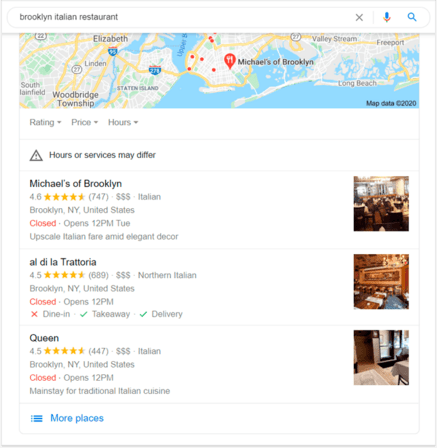The image depicts a screenshot of a cell phone actively using Google to search for "Brooklyn Italian restaurant." At the top of the screen, there is a horizontal rectangle displaying a map encompassing parts of New Jersey and New York, with a prominent red teardrop marker highlighting "Michaels of Brooklyn" in Brooklyn. Below the map, filters for "Rating," "Price," and "Hours" are available for refining the search results. A note indicates that the hours of service may vary.

In the search results, the first listing is "Michaels of Brooklyn," rated five stars. The restaurant is currently closed and scheduled to open at 12 p.m. on Tuesday. The next listed option is "Al Di La Trattoria," holding a rating of 4.5 stars. This establishment is also closed and will reopen at 12 p.m., located in Brooklyn. The final entry is "Queen," with a 4.5-star rating, also in Brooklyn, and currently closed with an opening time of 12 p.m.

Overall, the image offers a comprehensive overview of top-rated Italian restaurant options in Brooklyn, complete with ratings and operation hours.